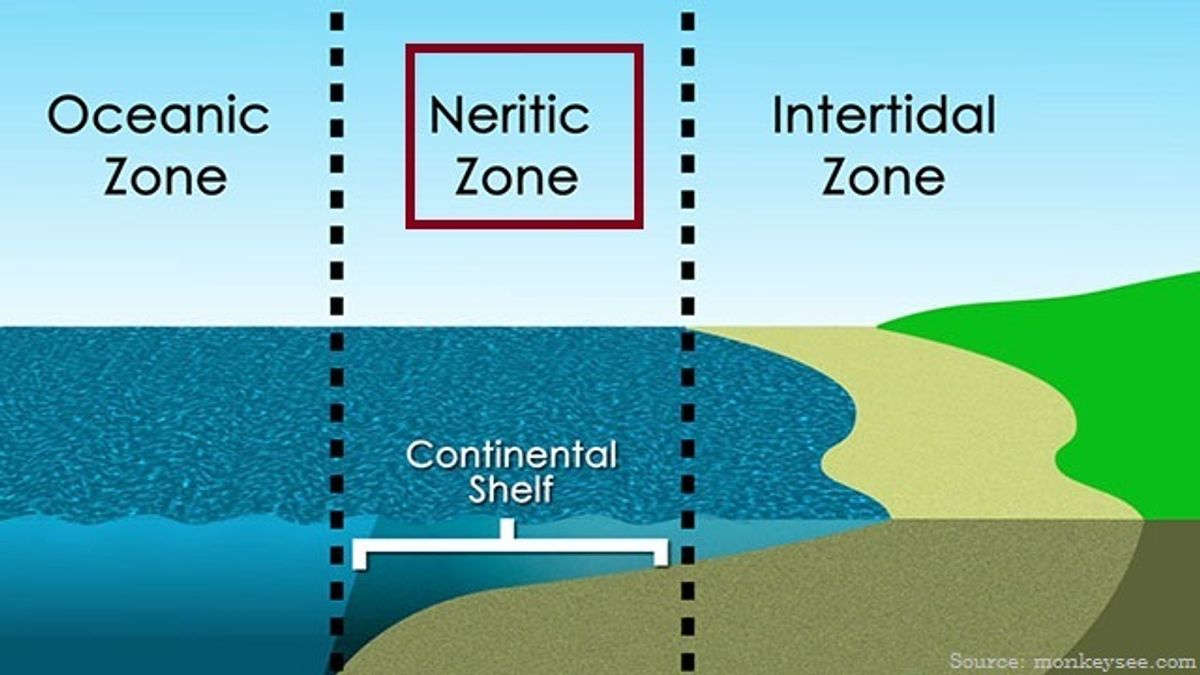This detailed illustration is split into three distinct sections with dotted lines and text labels set against a light blue sky background. The top-left corner reads "Oceanic Zone," indicating where the deep blue water of the ocean is located. The middle section, bordered in dark red, is labeled "Neritic Zone," with the text "Continental Shelf" beneath it and an arrow pointing to the underwater land drop-off. The final section transitions from a light brown beach to green grass, marked as the "Intertidal Zone." The chart is a rectangular, digital drawing sourced from Monkeysee.com, as noted in small white letters in the bottom-right corner.